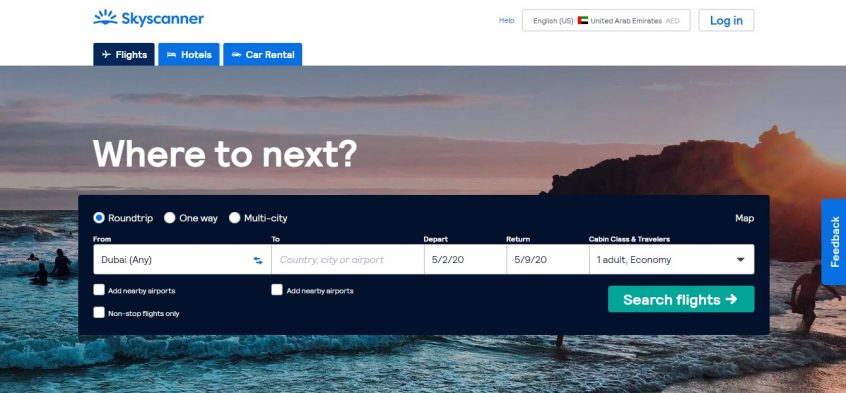The image showcases the Skyscanner website interface. In the top left corner, the Skyscanner logo and name are prominently displayed. On the right-hand side, there is a blue help menu, indicating the current language is set to English (US) and the country to the United Arab Emirates. To the right of these settings is a Login button.

Below the header, the site features several tabs for navigation: Flights, Hotels, and Car Rental, with the Flights tab currently selected, highlighted in dark blue. The main background image features a serene scene of people wading into the sea from a beach at sunset. Overlaying this image is the white text asking, "Where to next?"

Superimposed over the background is a blue floating panel with various flight search criteria. Users can choose between Round Trip, One Way, or Multi-City options, with Round Trip as the default selection. Additional fields allow users to specify departure and destination locations, departure and return dates, cabin class, and the number of travelers. Checkboxes give options to select non-stop flights only or include nearby airports.

At the bottom right of the blue panel is a green "Search Flights" button, ready to initiate the flight search process.